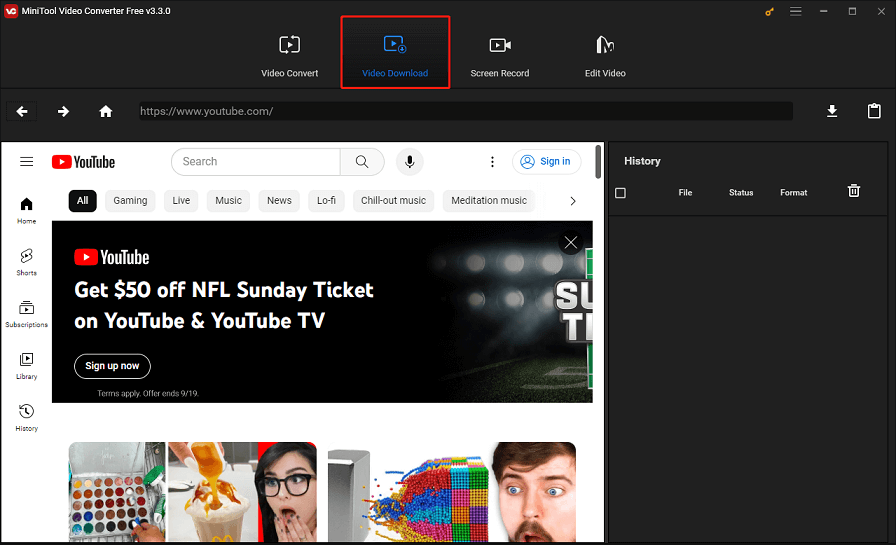This image is a screenshot from a website featuring the interface of MiniTool Video Converter Free, version 3.3.0. The background is predominantly black at both the top and right sides. In the upper left-hand corner, the text "MiniTool Video Converter Free" is displayed in white font, followed by "V 3.3.0". 

There is a top menu bar where various features are listed. Near the center, in blue font, it says "Video Download," accompanied by a blue square icon with a blue triangle pointing to the right, outlined in red. On the left side, the menu option "Video Convert" is written in white font, while on the right side, options for "Screen Record" and "Edit Video" are also present.

In the lower left-hand corner of the screenshot, a portion of the YouTube homepage is visible. This section has a white background with the familiar YouTube logo and name displayed prominently. Beneath the header, there are several category tabs such as "All," "Games," "Live," "Music," and "News." Below these tabs, an advertisement for the NFL Sunday Ticket is showcased, featuring a black background and white font with the text "Get $50 off NFL Sunday Ticket on YouTube and YouTube TV."